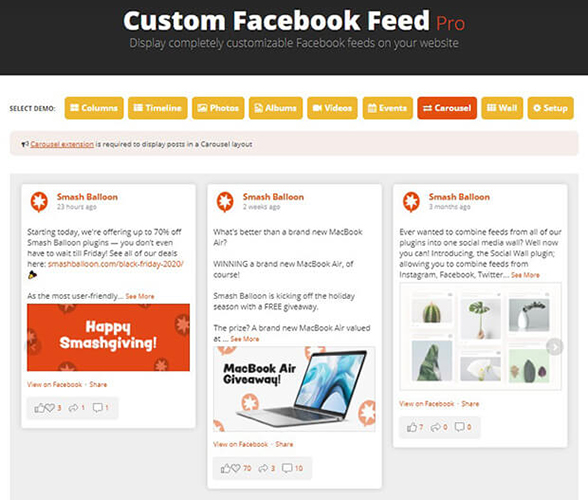This image features a promotional display for "Custom Facebook Feed Pro," highlighting its ability to seamlessly integrate fully customizable Facebook feeds onto your website. Across the top, bold text reads, "Display completely customizable Facebook feeds on your website," encapsulating the product's primary function. Below this header, to the left, there's a vertical menu titled "Select Demo," featuring various interactive yellow buttons. These buttons, listed horizontally from right to left and left to right, are labeled: Columns, Timeline, Photos, Albums, Videos, Events, Carousel, Wall, and Setup. Notably, the Carousel button stands out in red, indicating a distinct or highlighted feature.

Beneath the button menu, a series of example Facebook feeds are displayed, showcasing what the integration might look like in practice. Each feed example originates from a company called Smash Balloon and features a variety of posts, illustrating the diverse range of content and styles the plugin can accommodate.